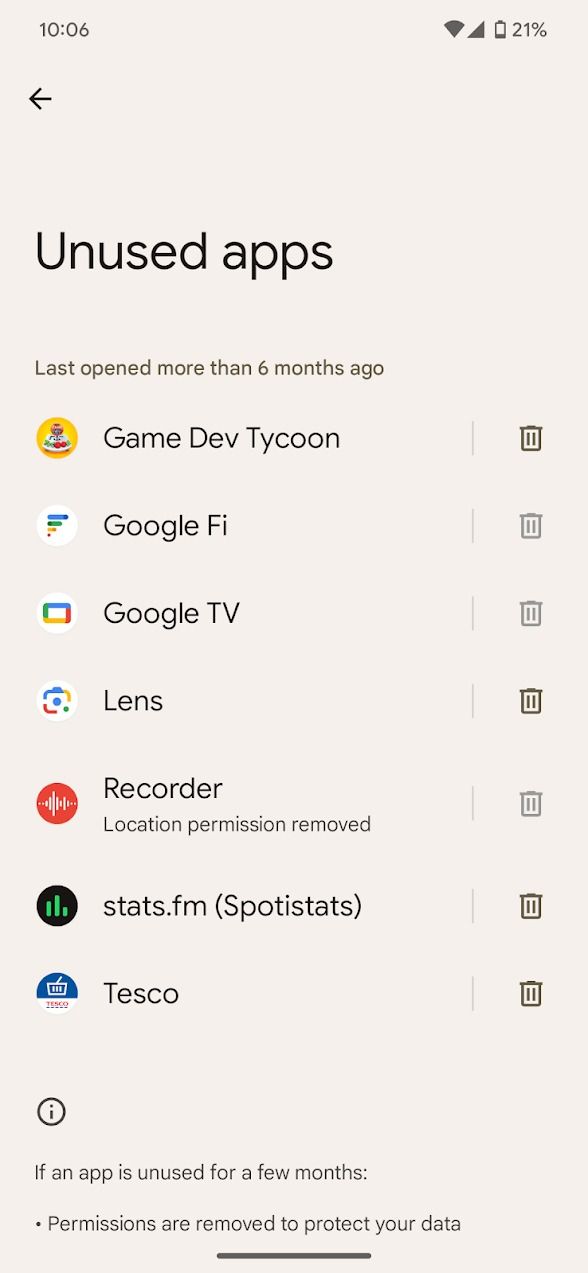A smartphone screen displays a list of unused apps, organized for potential deletion. The time is shown at the top as 10:06, with full Wi-Fi strength indicated next to a nearly depleted battery icon, displaying a charge level of 21%. A left-pointing back arrow is visible, alongside the heading "Unused Apps." Below this, it states, "Last opened more than six months ago."

The list of apps includes:
- **Game Dev Tycoon** accompanied by a trash can icon signifying the option to delete it.
- **Google Fi** with an adjacent trash can icon.
- **Google TV** with a trash can icon next to it.
- **Lens** followed by a trash can icon.
- **Recorder**, also paired with a trash can icon and a note that reads "Local permission removed."
- **Stats.fm Spot** and **Stats.fm** both with trash can icons.
- **Tesco** along with a trash can icon.

An information icon (a circled "i") appears at the bottom of the list. Additionally, a message at the bottom of the screen notes, "If an app is unused for a few months, permissions are removed to protect your data."